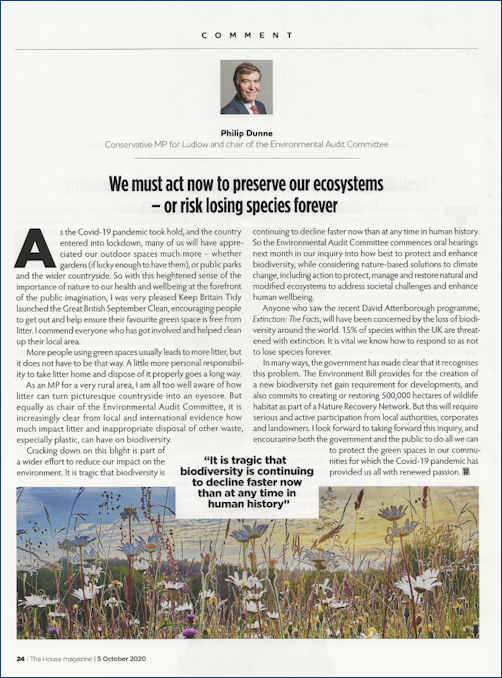Screenshot of a Digital Magazine Article

The image is a screenshot of a computer display showcasing a digital magazine article. The background is an off-white color with black text, giving the article a clean and professional appearance. The content includes a detailed article and two images.

At the very top center, the word "Comment" is prominently displayed, indicating the nature of the piece. Below it, there's a small profile picture of a man with brown hair wearing a blue suit jacket and a red tie. He is identified as Philip Dunn, a Conservative MP for Ludlow and Chair of the Environmental Audit Committee.

The article is titled, "We Must Act Now to Preserve Our Ecosystems or Risk Losing Species Forever," and it emphasizes the urgency of environmental conservation. The text is divided into two rows: the first row contains four paragraphs, while the second row consists of two paragraphs. 

Interrupting the flow of the second row of text is a pop-up rectangle featuring a poignant quote: "It is tragic that biodiversity is continuing to decline faster now than at any time in human history."

At the bottom, there is a large picture depicting vibrant flowers set against a blue sky, visually reinforcing the article's environmental theme. The page number "24" and the date "5 October 2020" are visible at the very bottom of the image, signifying the article's placement and date of publication.